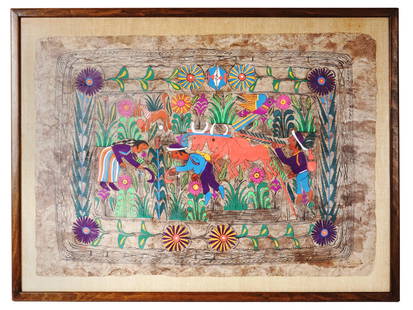This image features a detailed painting depicting a scene of three individuals, likely Native Americans, engaged in gardening within a vast array of colorful flora. The painting is enclosed in a rustic, dark brown frame, with an outer frame of light brown. Vines and flowers border the painting, featuring purple flowers in each of the four corners, connected by leafy chains and wheel-like designs with orange centers.

The vibrant scene at the center shows three figures: one person standing on the right, possibly holding a branched instrument, and two others bent over, planting seeds on the left. They are surrounded by a rich tapestry of flowers in hues of pink, orange, yellow, and purple, set against lush greenery. A clear patch of brown soil in the middle highlights their gardening activity. The top and bottom of the painting mirror each other, with similarly patterned floral designs and more purple flowers at the corners, completing the harmonious composition.